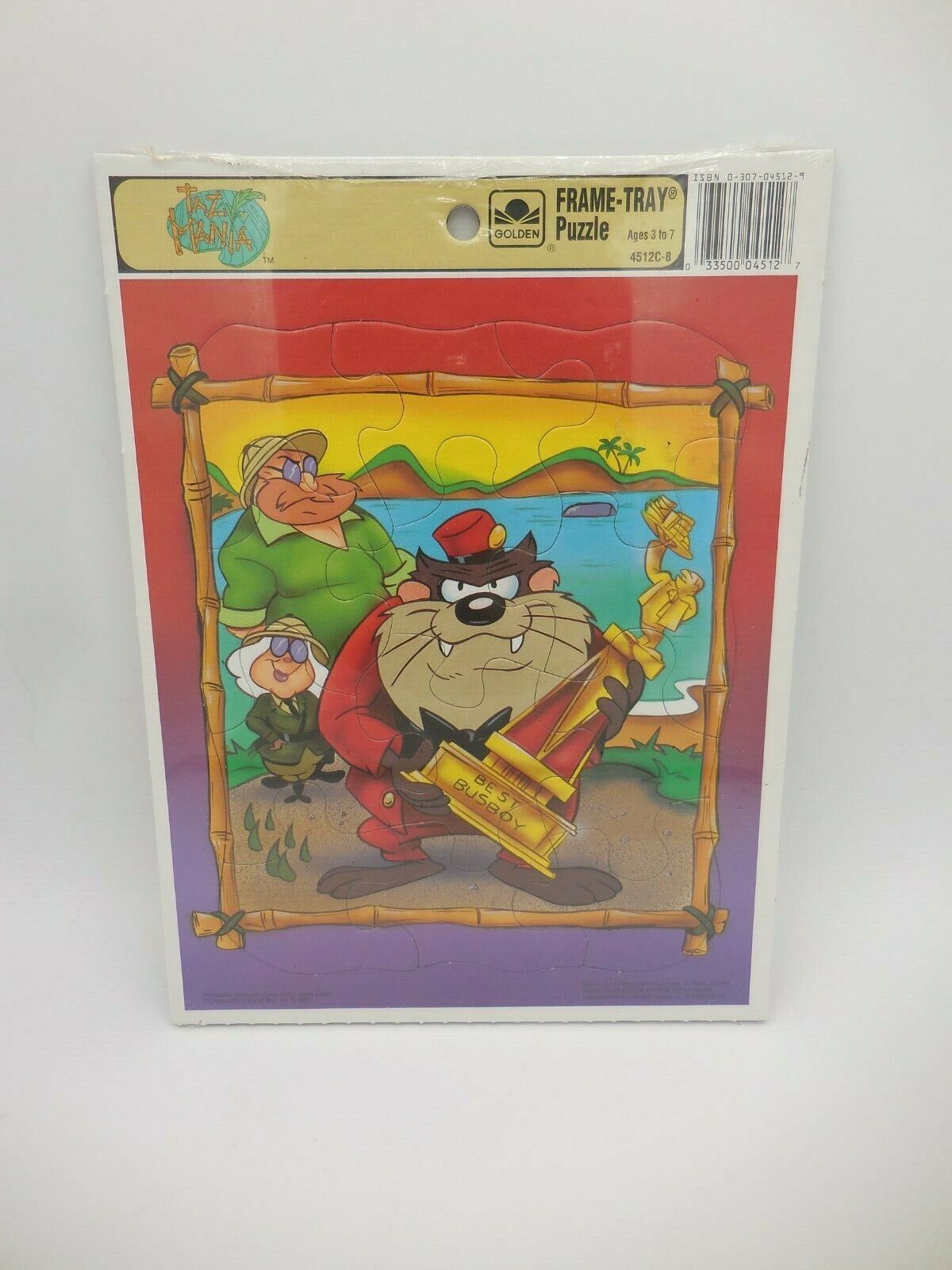This full-color photograph portrays a cardboard frame tray puzzle designed for young children, featuring a vividly illustrated scene from the show *Tasmania*. The vertically rectangular image shows no border or additional background beyond the puzzle itself. At the top, there is a punched hole meant for display on a rack. The puzzle's surrounding edge is made to resemble bamboo framing, detailed in tan and red.

Central to the illustration is the Tasmanian Devil dressed in a red bellhop suit with gold trim, holding a golden trophy that reads "Best Busboy." Standing behind him are two characters in safari gear: a much larger, full-bearded man in a green shirt and tan pith helmet, and a significantly shorter woman with white hair also in a pith helmet, donning a dark green jacket and tie. Both characters wear glasses.

The background showcases a tropical landscape, complete with blue waters, islands, palm trees, and a gradient sky transitioning from red to purple. The beach scene offers a vibrant and engaging setting that is likely to appeal to children.